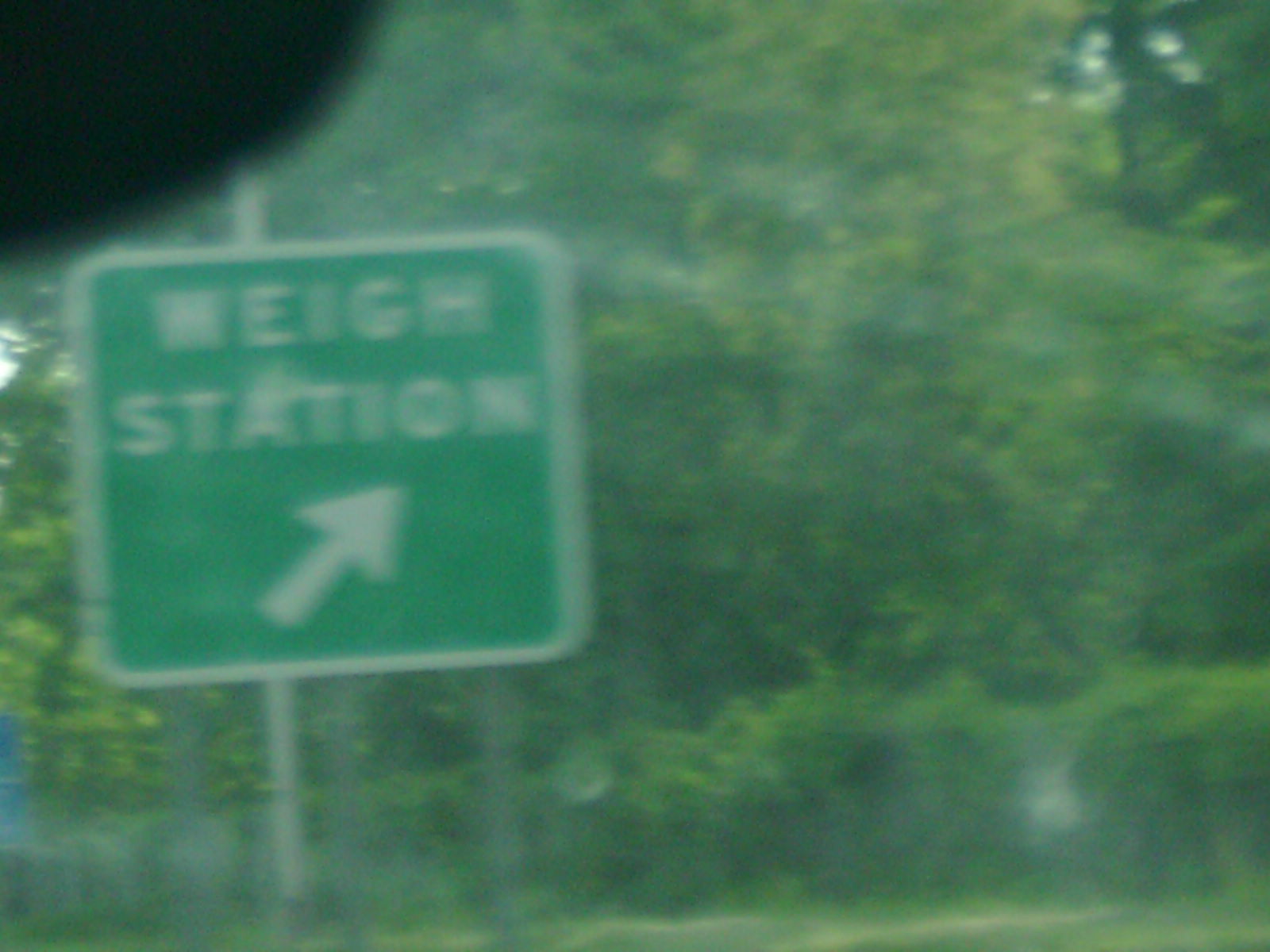A blurry photograph taken from the window of a moving car, capturing the scene through spotty and unclean glass, creating a white haze over the image. The photo prominently features a large square green road sign with a white border occupying approximately half of the frame on the left side. The sign, supported by three gray posts and a white lamppost behind it, reads "Way Station" with an arrow pointing diagonally up to the right. Surrounding the sign is a grassy area with tall green bushes and trees in the background. A noticeable black spot is present in the top left corner of the photograph.